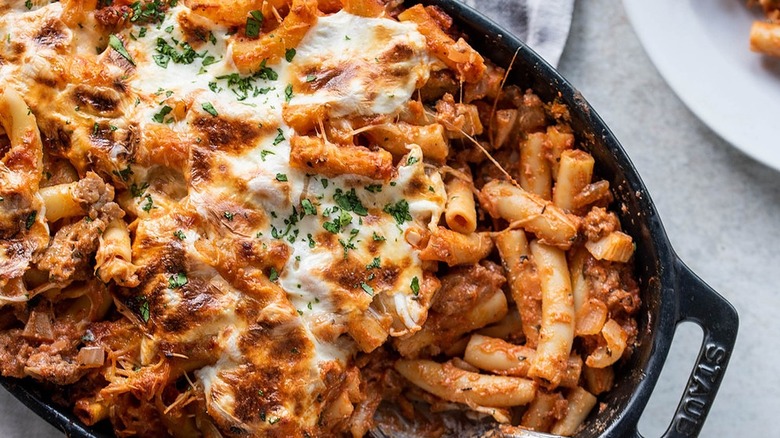This detailed, close-up, overhead shot captures a delectable rigatoni pasta dish served in a black cast iron Staub oval pan. The tubular rigatoni is generously coated in a rich tomato sauce, which seems to contain bits of meat and onions. The dish is topped with broiled, lightly browned melted cheese, creating an enticing cheesy pull effect, and is garnished with a sprinkling of fresh parsley. The pan sits atop a grey countertop. In the top left corner of the image, a sliver of a whitish grey plate is visible, while the top right corner shows a white plate with a serving of the rigatoni. The photo evokes the essence of dining at a restaurant, capturing the vibrancy and richness of the pasta and its carefully baked, aromatic topping.